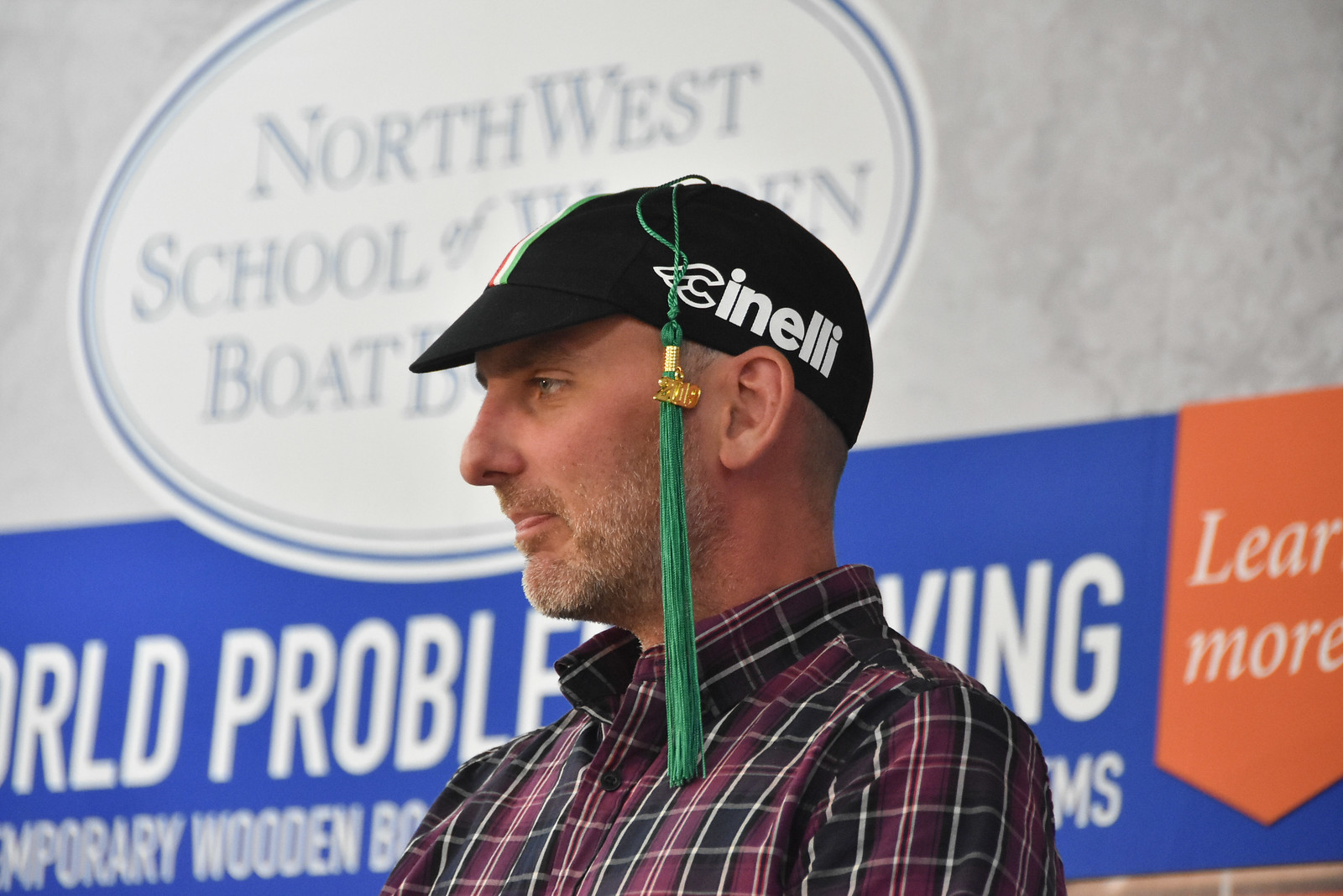The photograph captures a man from his lower shoulders to the top of his head, with his body and face turned towards the left of the frame. He is wearing a black, purple, and white plaid shirt with black buttons, leaving the top button at the collar undone. His light blonde and gray stubble accents his cheeks, chin, and lip, which is slightly open as he licks his lips with his pink tongue. A black baseball cap adorned with white text reading "Cinelli" and a green graduation tassel with a gold pendant adorns his head. Behind him, a large billboard partially reads "Northwest School of Western Boat," with additional, obscured text beneath it. Some of the visible lettering on the sign includes parts of phrases like "world problem solving" and "learn more," along with hints of other words and logos that remain partially hidden by the man's presence in the foreground.